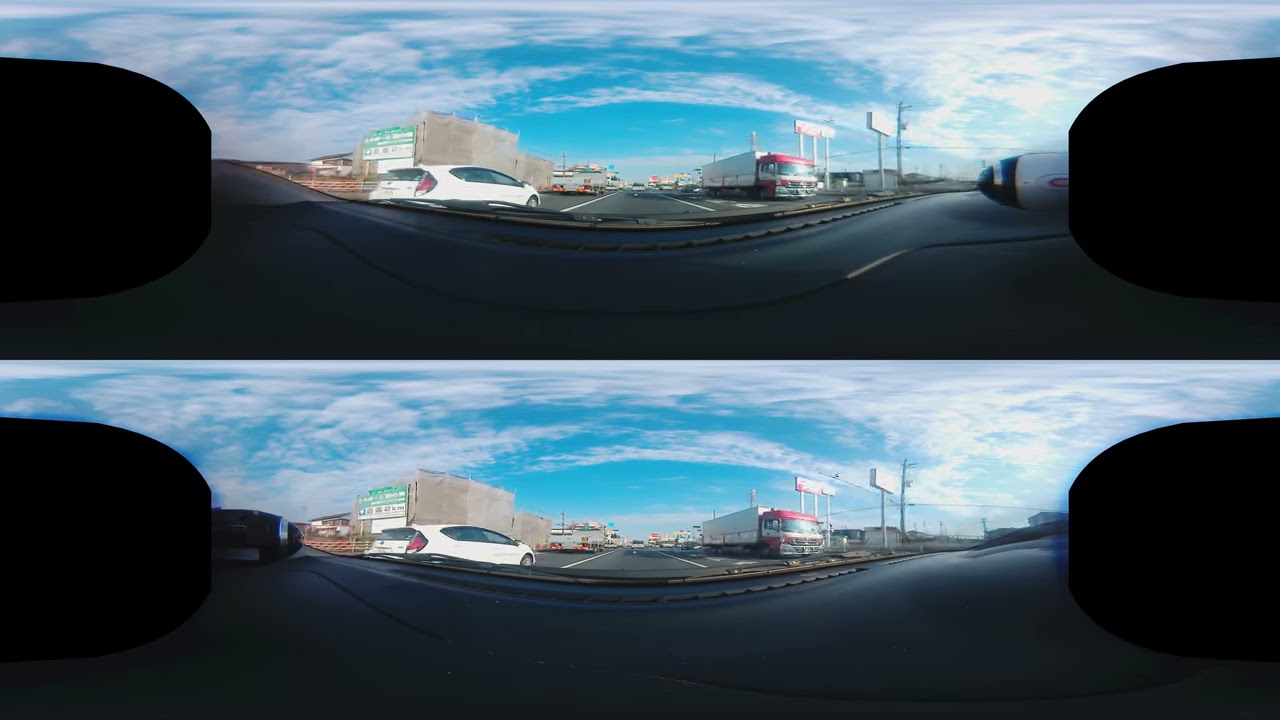The photograph, captured with a fisheye lens, presents a surreal, panoramic view from inside a car, likely from the back seat, given the visible headrests and absence of windshield wipers. The image is uniquely split in two, with an identical replica placed below the original. The curved perspective frames a freeway scene, showing a central road flanked by two lanes moving in opposite directions. 

To the right, a menacing red 18-wheeler with a gray trailer advances toward the viewer, while a white car on the left heads away. Enclosing the scene are large, dark shapes on either side, potentially the car’s seats or interior framework. 

Blue sky filled with scattered white clouds arches overhead, while in the background, indistinct buildings and various billboards create a vague urban landscape. Additional roadside signs perched on tall poles can be seen on both sides of the road, enhancing the depth of this dynamic, mirrored image.